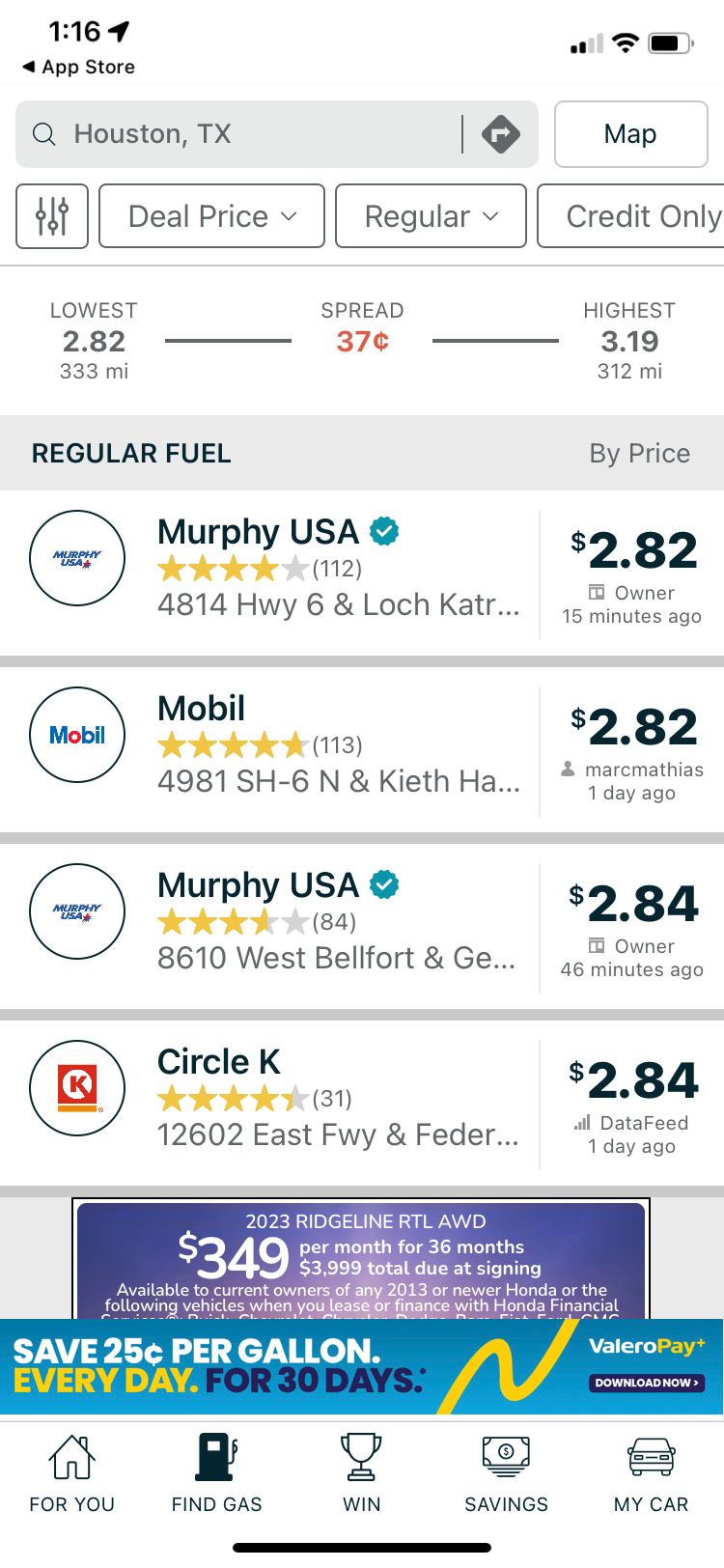The image displays an interface of a gas station app designed to assist users in finding the best gas prices in their vicinity. At the top of the app, there are options for inputting the city and state, along with directions to the selected gas station. The app provides various map options and detailed pricing categories, including deal prices, regular options, and credit-only options. It showcases a price range, with the lowest price listed at $2.82 and the highest at $3.19, indicating a price spread of $0.37. 

The app highlights which gas stations offer the cheapest gas, with ratings and prices given as follows:
- Murphy USA: $2.82 (4 stars)
- Mobile: $2.82 (5 stars)
- Murphy USA: $2.84 (4 stars)
- Circle K: $2.84 (4.5 stars)

At the bottom of the app, advertisements are displayed, including an offer for a 2023 Ridgeline RTL all-wheel drive at $349 per month for 36 months. Additionally, there's a promotion from Valero stating "Save 25 cents per gallon every day for 30 days" with instructions to download the associated app. Finally, navigation tabs for "Find Gas," "Win," "Savings," and "My Car" are noted at the bottom of the screen.